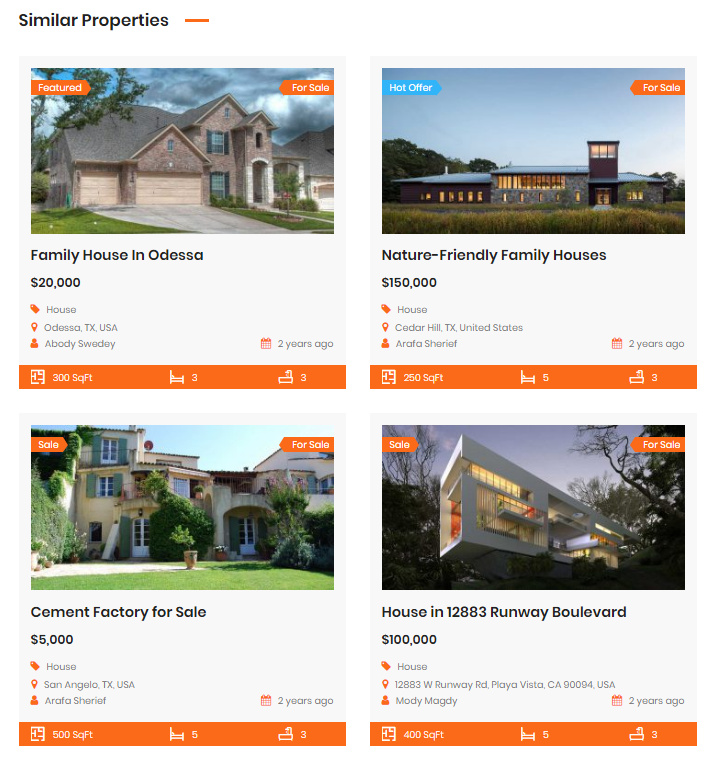This screenshot depicts a search results page from a real estate website showcasing four houses, each accompanied by a photograph and detailed information. 

1. **House in Odessa, Texas:**
   - **Status:** Featured for Sale
   - **Price:** $20,000
   - **Type:** Family House
   - **Location:** Odessa, Texas
   - **Details:** Listed as 300 square feet, though the image suggests a much larger property, likely around 2,000 square feet.
   - **Additional Info:** Sleeps three; listed two years ago by an entity labeled "a body, sweetie."

2. **Nature-Friendly Family House:**
   - **Status:** Hot Offer for Sale
   - **Price:** $150,000
   - **Type:** Family House
   - **Description:** Described as only 200 square feet, but the photo shows a large mansion, potentially around 5,000 square feet.
   
3. **Cement Factory (San Angelo, Texas):**
   - **Price:** $5,000
   - **Type:** Cement Factory (though visually contradictory with the photo of a beautiful tropical mansion)
   - **Location:** San Angelo, Texas
   - **Listed by:** Arafa Sharif
   - **Details:** Noted as 500 square feet.

4. **House on 12883 Runway Boulevard:**
   - **Price:** $100,000
   - **Type:** House
   - **Location:** 12883 Runway Boulevard
   - **Description:** Mountain-crested house with numerous windows and scenic valley views; visually resembles a million-dollar property.
   - **Details:** Listed as 400 square feet; noted by Mahdi Magdi two years ago.

All property pictures appear to conflict with their respective descriptions, suggesting possible listing errors.